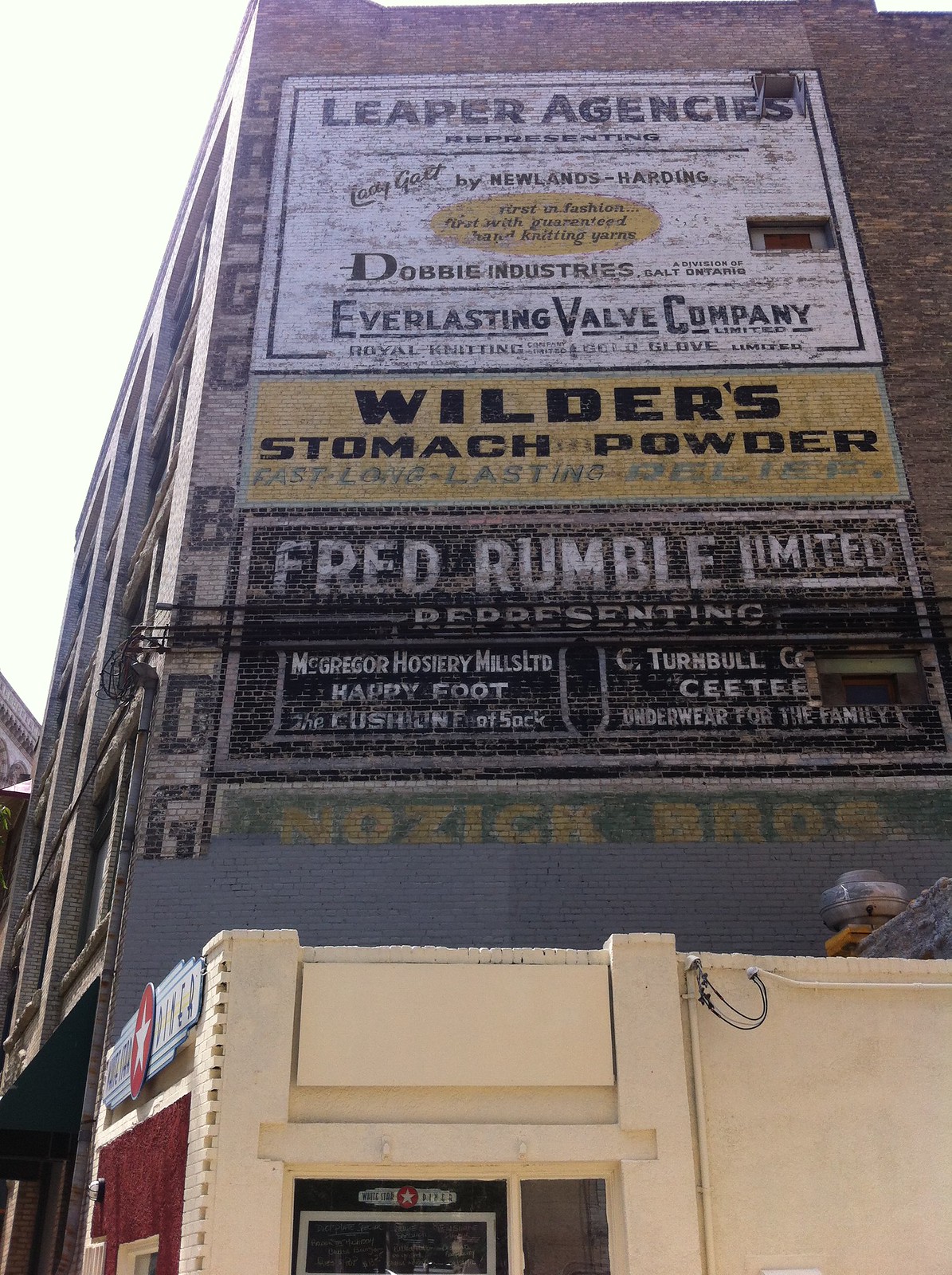The image depicts an outdoor scene showcasing the side wall of a large, old brick building adorned with a series of vintage-style painted advertisements. Prominently displayed on the wall are the following advertisements: "Leaper Agencies," "Everlasting Valve Company," "Wilder Stomach Powder – Fast, Long-lasting Delivery," and "Fred Rumble Limited."

The text on the wall also references companies such as "Dobby Industries," "McGregor Hosiery," and "My Mills LTD." Painted with a variety of colors including white, brown, gray, yellow, black, green, maroon, and light blue, these advertisements span the height of the wall, giving it an aged, rustic appearance.

At the bottom of the image, a small white diner with a star in its signage is visible, situated at the base of the building's wall. The setting is outdoors in the middle of the day, suggesting a bright and clear atmosphere. The image is centered on the building, capturing a snapshot of a historical and charming urban landscape.